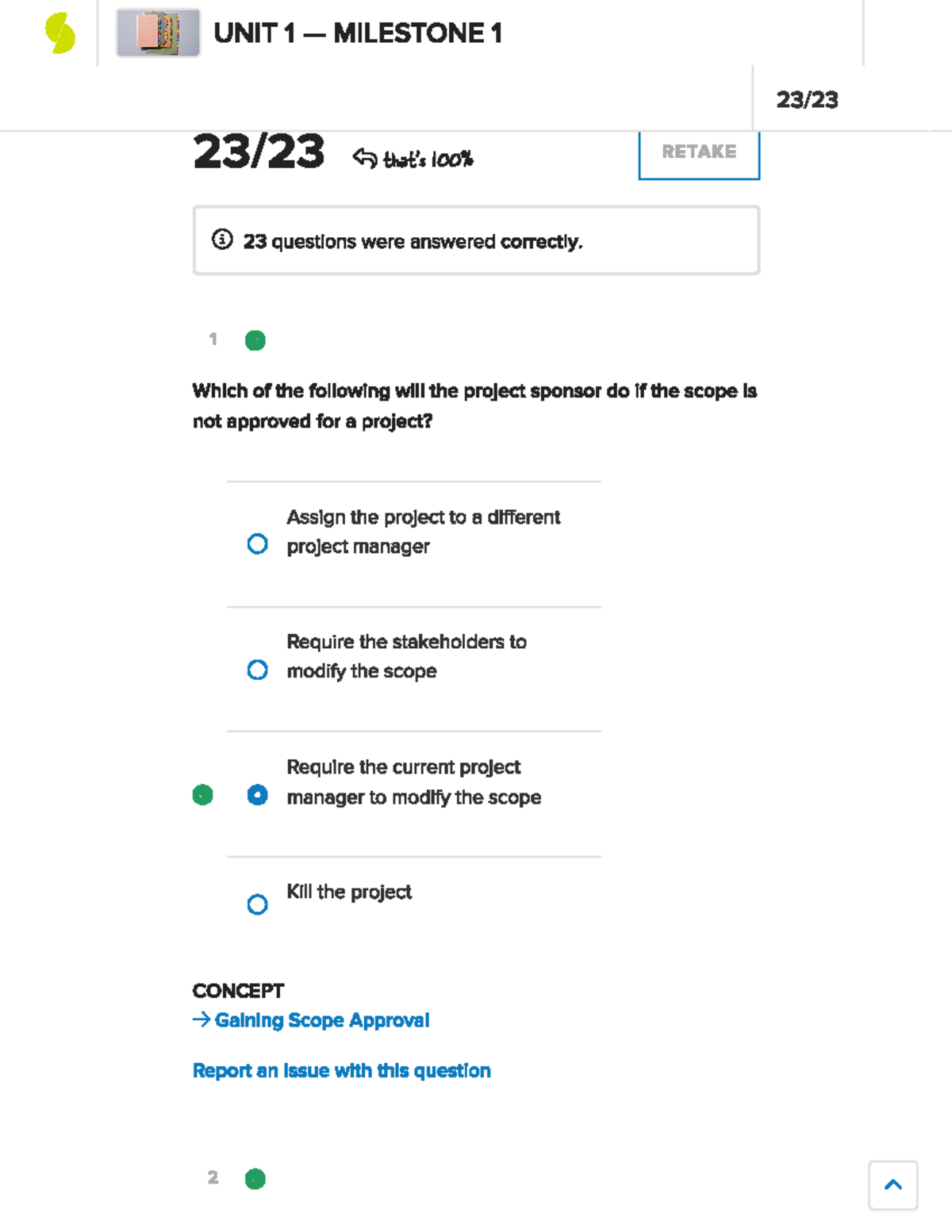**Webpage Description:**

At the top left corner of the webpage, there is a forest green symbol resembling a halved circle with one piece sliding above and the other below. On the top right, there's a dark grey square featuring stacks of multicolored papers in pink, blue with red and blue accents, orange, and forest green with some red highlights. To the right of this section, bold black text reads "Unit 1 - Milestone 1," and adjacent to it is a completion indicator "23/23," signaling that all 23 items have been completed, with "23 out of 23" reiterated in bold black text. A thin grey line precedes this text before it switches back to black and bold, with an arrow pointing towards it and a note stating "100%" as if edited into an image.

To the right, there's a button with a blue border and grey text labeled "retake." Below this button, a lighter grey-bordered rectangle features an information bubble on the left, depicted as a circle with an eye icon. Bold black text within this rectangle declares, "23 questions were answered correctly," followed by a dark grey number "1" and a green circle with a grey checkmark.

In the next section, a question asks, "Which of the following will the project sponsor do if the scope is not approved for the project?" There are four answer choices, with the third one selected and marked correct — a dark blue circle with a white checkmark inside a green circle indicates: "Require the current project manager to modify the scope." The other options—"Assign the project to a different project manager," "Require the shareholders to modify the scope," and "Kill the project"—are in bordered blue circles with white interiors.

At the bottom of the page, bold black text reads "Concept," followed by a hyperlinked arrow pointing right to "Gaining scope approval," and an option to "Report an issue with this question." Below this, a grey number "2" is shown next to a green circle with a grey checkmark, and on the far right, a muted grey square with a blue arrow pointing up is displayed.